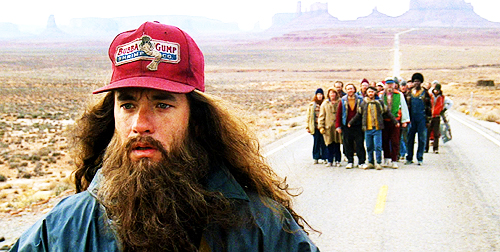In this daytime scene from the movie "Forrest Gump," Forrest Gump, played by Tom Hanks, is shown in the midst of one of his long runs. He stands still, having stopped in the middle of an open, wide landscape. Behind him, a group of about 50 runners is also pausing. Forrest is distinguishable by his long hair, bushy beard, and the iconic red "Bubba Gump" hat. He is wearing a running jacket over a blue jean shirt, and a perplexed yet serious expression adorns his face, indicated by his furrowed eyebrows. In the far distance, the Utah Plateau Mountains provide a majestic backdrop to the scene.